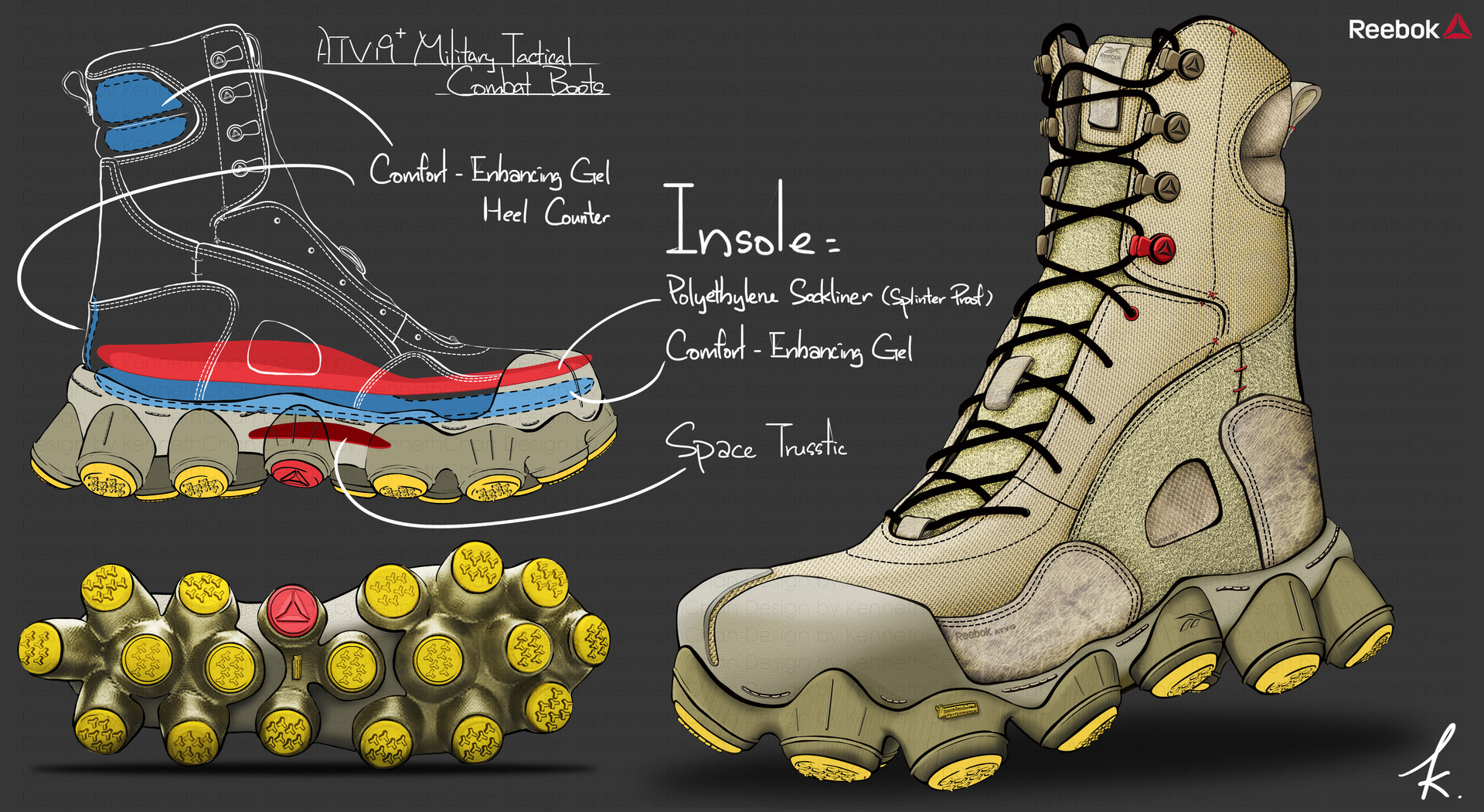This mockup illustrates a detailed design of Reebok's ATV19+ Military Tactical Combat Boots. In the upper right corner, the Reebok logo is prominently displayed beside a red triangle. The bottom right corner features a distinct letter "K." Central to the image is a cutaway view of the boot, highlighting its internal features, including Comfort Enhancing Gel, Heel Contour, Insole, Polyethylene construction, and a Sock Liner (with text in parentheses that is too small to read). Also noted are the terms Comfort Enhancing Gel and, presumably, "Spacetrustic." The bottom section of the boot showcases a sole comprised of numerous cleat-like structures, presumably for superior traction. In addition, a full view of the boot reveals its color scheme—light shades of green with a yellow outsole, further emphasizing its rugged, tactical aesthetic.